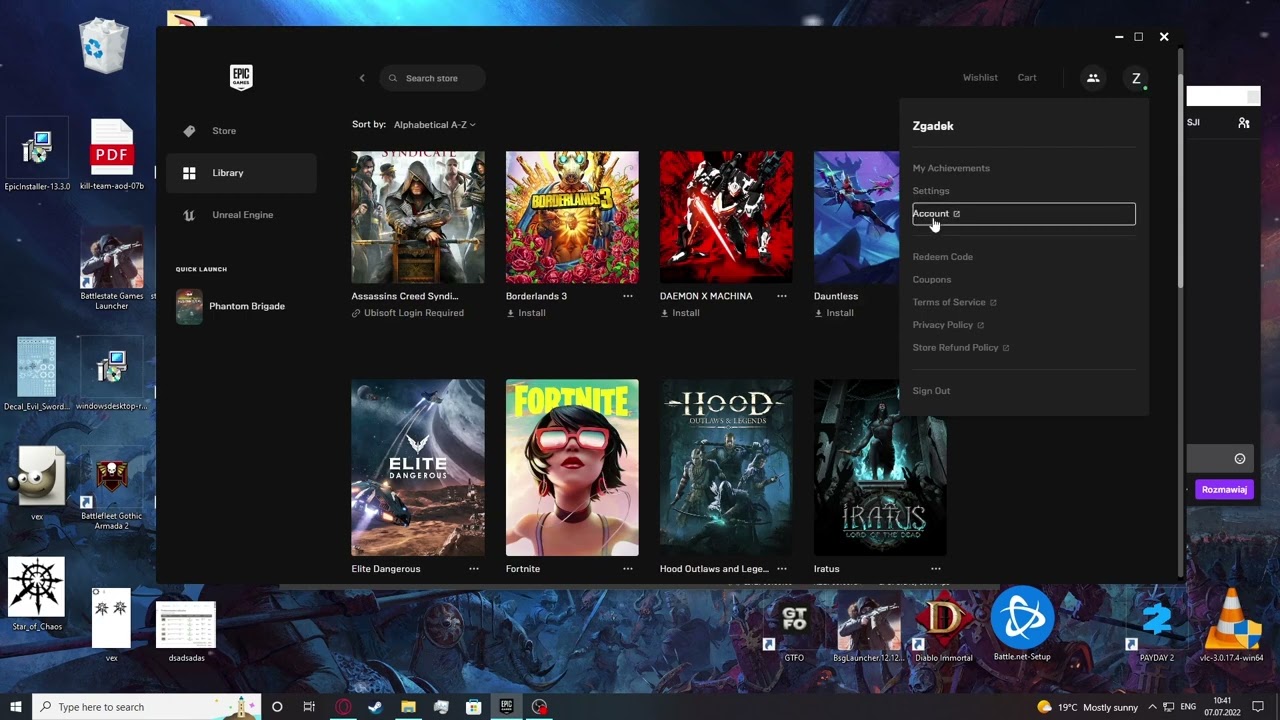The screenshot displays a cluttered desktop on a Windows computer. The desktop wallpaper sets a fantastical scene, bathed in various shades of blue, depicting a peculiar animal with a saddle and a rider navigating through the fantasy landscape. 

Several icons are scattered across the desktop, somewhat obscuring the enchanting wallpaper. At the bottom of the screen, the Windows taskbar is visible, featuring a white Windows icon composed of four squares on the left, next to a search field with a black magnifying glass labeled "Type here to search." To the right, there's a small cartoon icon typical of Microsoft's style, but its details are indistinct.

Open applications crowd the screen; visible are the windows for Steam, a file explorer, the Microsoft Store, and the Epic Games Store. In the lower right corner, the system tray displays the current temperature as 19°C and the time, although the time is too small to be legible.

The foreground prominently features the Epic Games Store window, which is black and showcases the user's library of games.